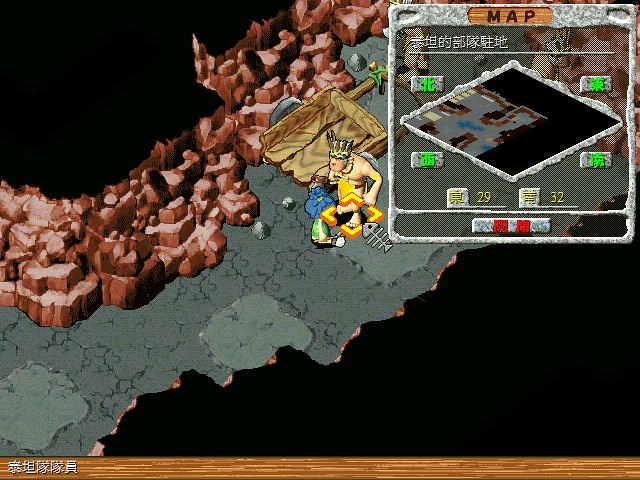This screenshot from a video game depicts a central character with peach skin, adorned in a gold and yellow loincloth, and a gold band around his right arm. He wears a feathery cap that is brown and gray with a yellow, black-spotted bandana. The character is located in a cave-like area, surrounded by dark and light brown rocks on both sides. The ground beneath him is a mix of dark and light gray, with the light gray sections forming small, rounded squares. A noticeable feature nearby is a dead fish skeleton. To the left of the character stands a smaller figure with blue hair, a dark green shirt, and pale skin, next to a light brown wooden wagon with dark gray zigzag patterns. On the right side of the screen is a topographical map of the area, with dark corners and sections of the display that appear to be partially obscured. The screen also shows bright green symbols on a gray background in each corner and yellow symbols with numerals "29" and "32" at the bottom, written in kanji. The main character, depicted with a yellow crown and a golden beard, stands under a glowing yellow cursor highlighting his position.